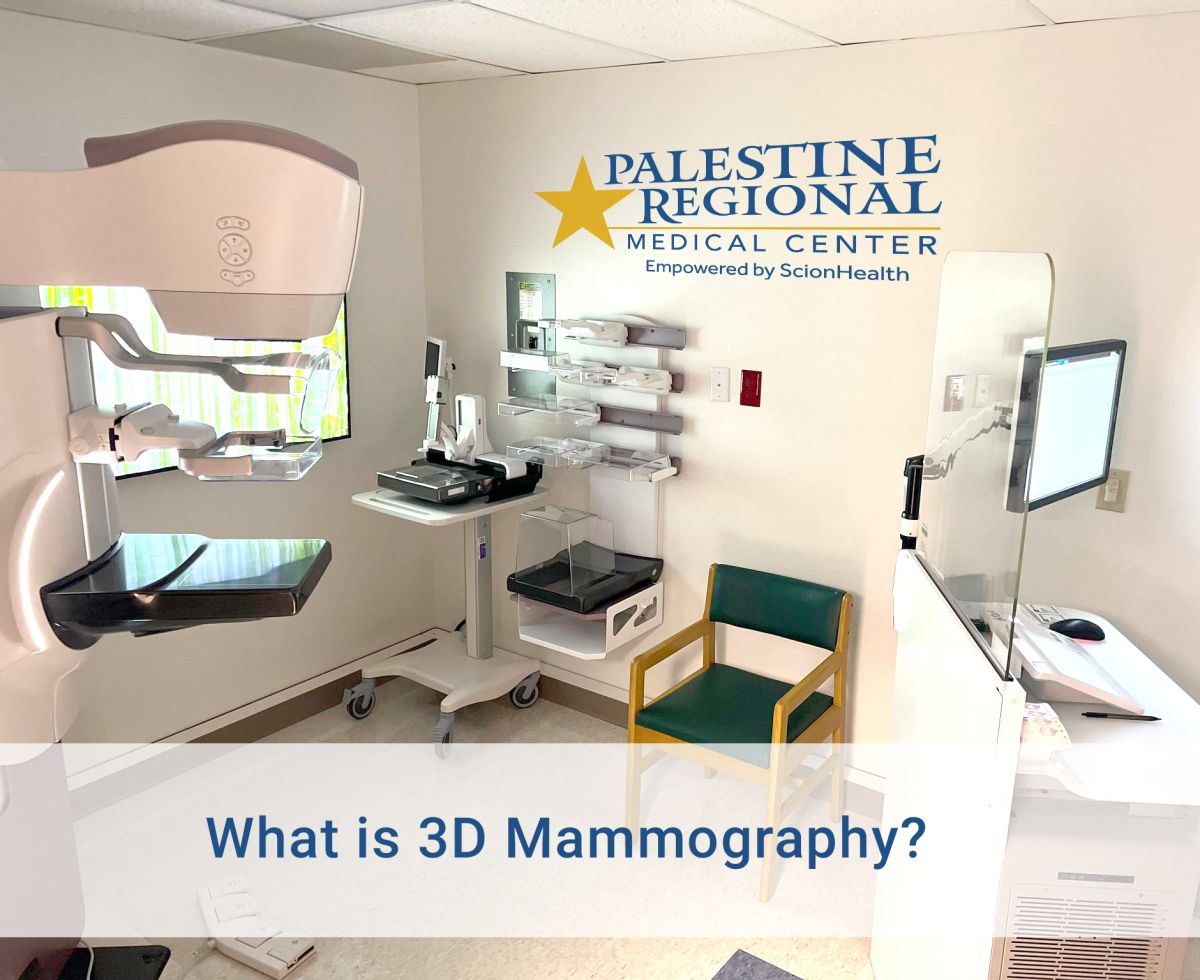The photograph depicts a room inside the Palestine Regional Medical Center, empowered by Scion Health, as indicated by the large blue text and gold star on the far wall. The room houses various moderately new medical and electronic equipment, including a mammogram machine on the left side and a rollie computer kiosk on a wheeled cart. On the right side, there is a computer desk surrounded by a glass shield, a typical feature in radiology environments. A small wooden chair with a padded green backrest and seat cushion is stationed against the far wall under the sign. Additionally, the bottom of the image features a semi-transparent white bar with blue text that reads, "What is 3D mammography?" This room appears equipped for conducting 3D mammograms and other medical procedures.